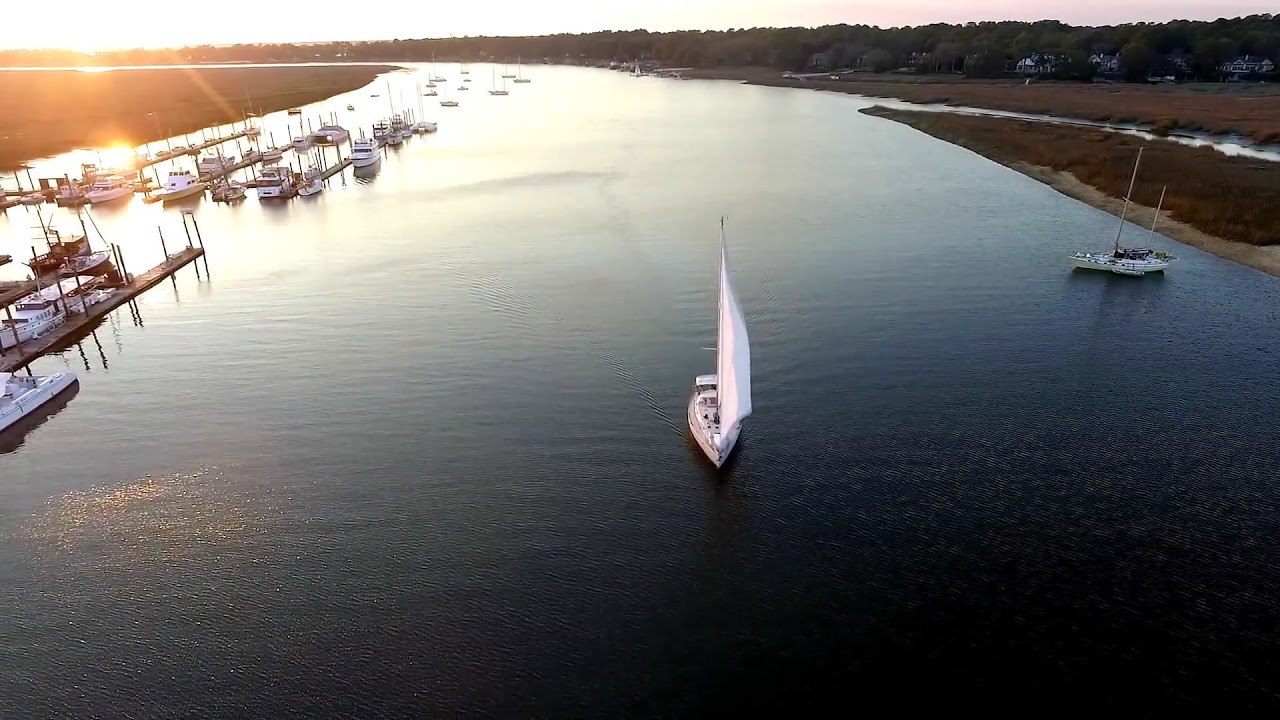The image captures a vibrant overhead view of a river bathed in natural daylight. The serene blue water of the river reflects the sky above and is dotted with several boats. In the center, a striking white sailboat with its large sail unfurled is navigating directly towards the photographer, its pristine white color contrasting with the darkening hues of the water. To the boat's right, another smaller vessel is visible, though it lacks sails. On the left side, the river is lined with docks and piers, where numerous other boats are moored. Both shores of the river offer different vistas: the left shore is an active dock area, while the right shore is lush with grass and dotted with houses nestled among trees, providing a picturesque backdrop. The top left corner of the image is illuminated by the bright, sparkling light of the setting sun, its brilliance mirrored in the water below, giving the scene a sprinkling effect. This detailed, color image encapsulates the tranquility and activity of a riverside setting, absent of any people or textual elements, capturing a moment where nature and nautical life coexist beautifully.